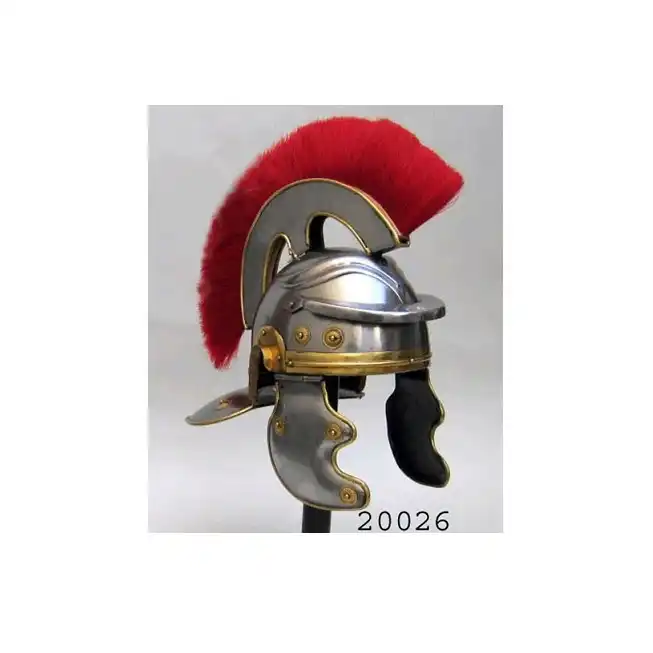This image features a detailed photograph of a helmet, resembling the style of a Roman Legionnaire's helmet. The helmet itself, oriented almost straight on but slightly from the side, is crafted from a silver-colored metal with gold accents, notably on the front headband and rivets. Distinct metal flaps hang down over the ears, also adorned with intricate gold detailing. Atop the helmet sits a striking red crest, reminiscent of a giant red mohawk, suggesting both ceremonial and decorative use. The image includes the numbers "20026" at the bottom, which might indicate a reference or lot number, adding to the impression that this could be a stock photo intended for cataloging or auction purposes. The overall color palette includes shades of silver, gold, red, black, gray, and white.